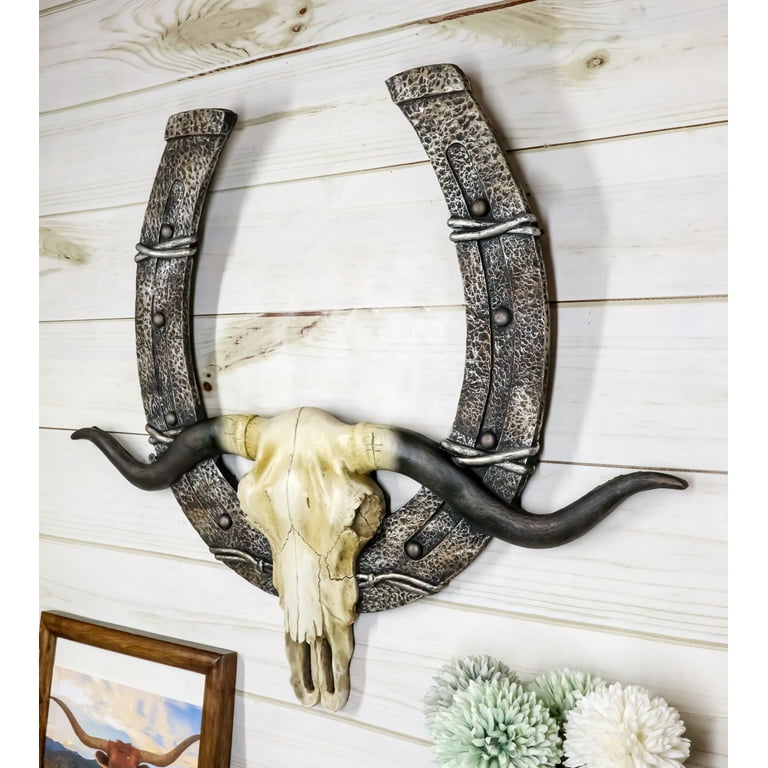The photograph captures a rustic or cabin-like setting, focusing on a white horizontal wooden plank wall, adorned with knots and colorations. Centered on the wall is a large, black and silver metal horseshoe, detailed with screws for an authentic effect. Suspended from the bottom of the horseshoe is a bleached off-white cattle skull featuring long, wavy black horns. Below the horseshoe, in the bottom left corner, is a framed picture displaying the top of another cow's horns, set in a brown frame. In the bottom right corner, a cluster of artificial flowers, including white and light green ones, add a soft touch to the composition.